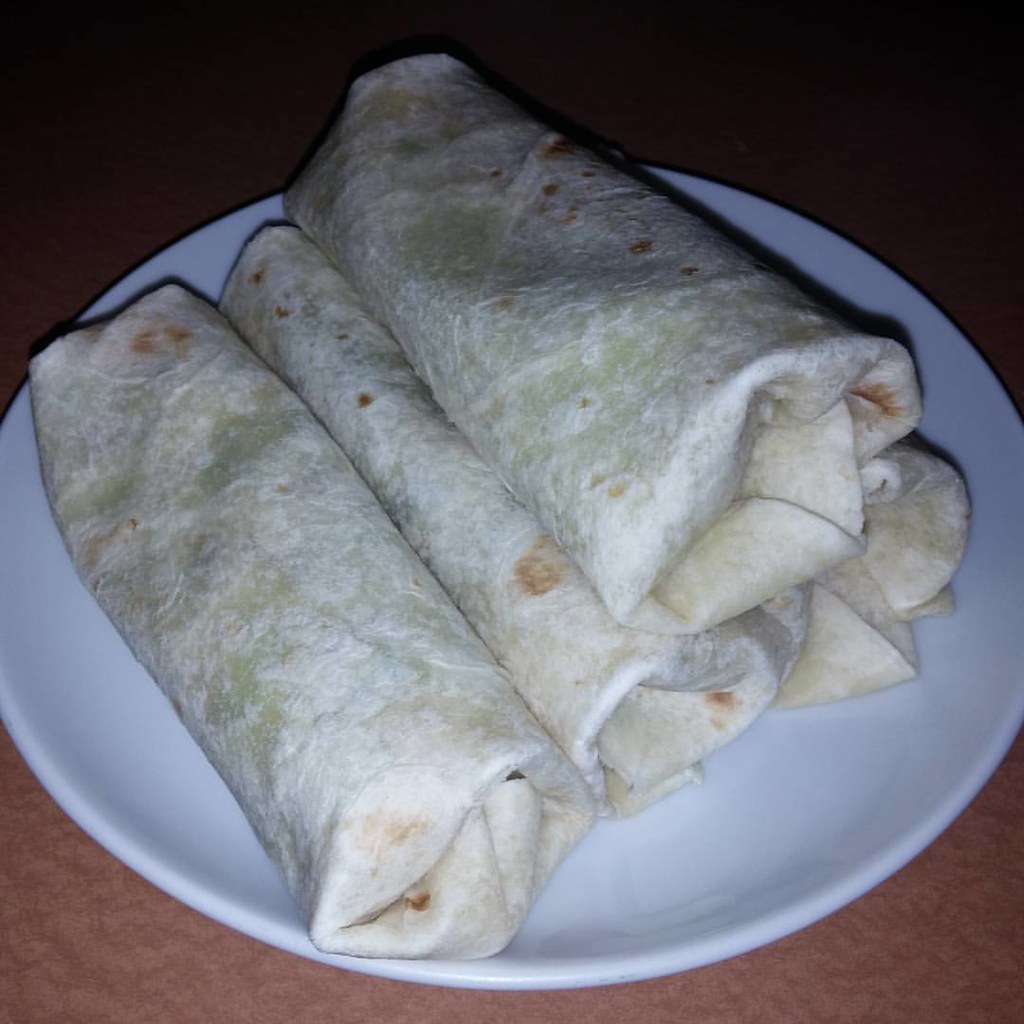In this detailed up-close photograph, a white plate sits on a table, possibly light pink or brown in color, with a black background in the upper corners of the image. Four large burritos, their flour tortillas lightly speckled with brown spots, are arranged on the plate. Three burritos lie side by side on the bottom, while one rests on top, straddling two of the burritos underneath. The tightly-wrapped burritos are sealed at the ends to hold in their filling, though none of the contents are visible. The thick, round burritos suggest they are quite filling, making a substantial meal.